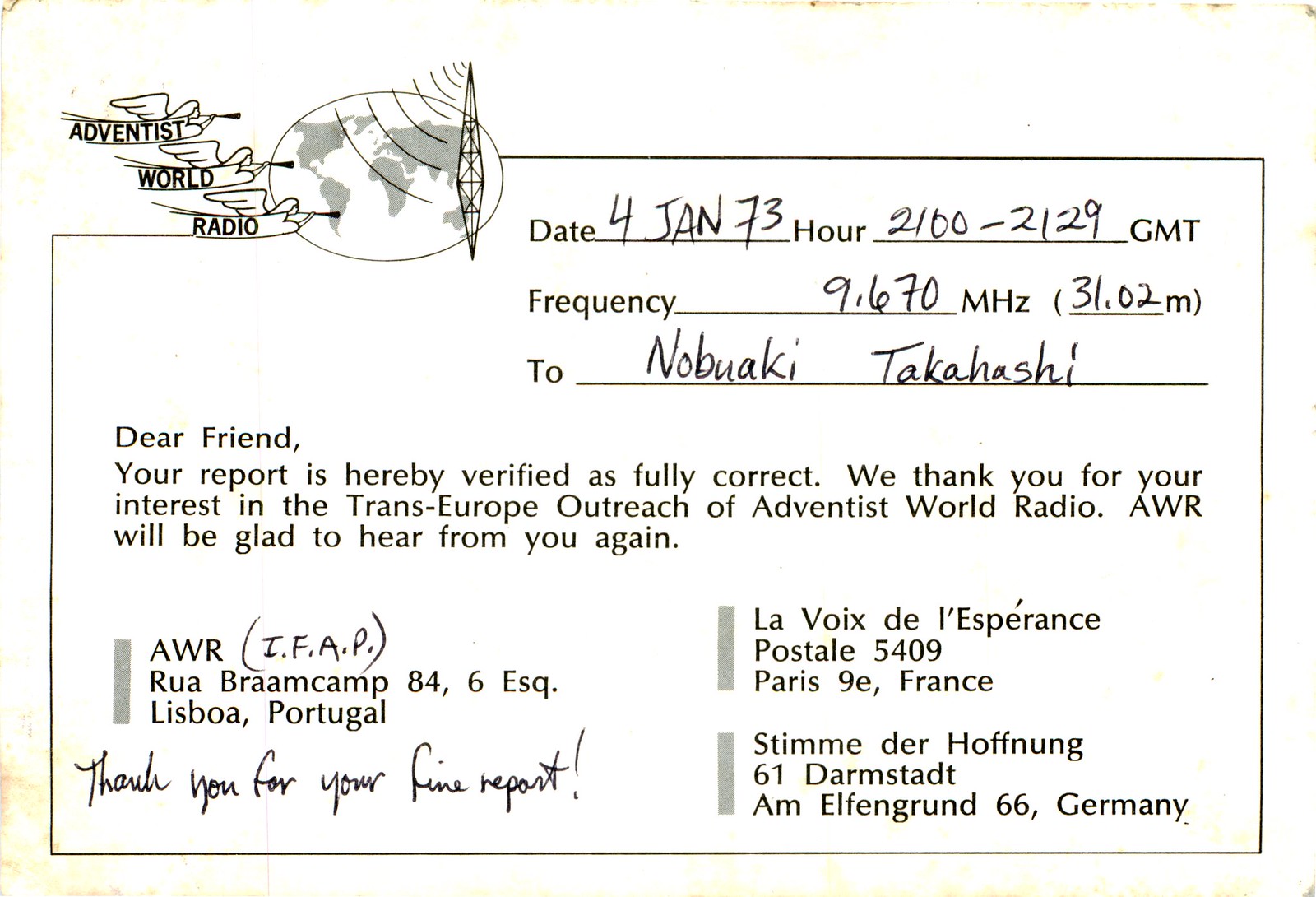This is an image of a vintage postcard, notably yellowed with age and featuring red stains along the edges. The postcard, centered around Adventist World Radio, prominently displays their logo in the upper left—a black and white sketch of a globe with wireless signals emanating from a tower, accompanied by three simple angels blowing horns. The text includes administrative details: date "4 Jan 73," time frame "2100 to 2129 GMT," and a broadcast frequency of "9.670 MHz, 31.02 M." Addressed to Nobuaki Takahashi in handwritten script, the letter reads: "Dear friend, your report is hereby verified as fully correct. We thank you for your interest in the Trans-Europe Outreach of Adventist World Radio. AWR will be glad to hear from you again." Additionally, the bottom left of the postcard provides the address "Rua Bramkamp 84, 6 Esq., Lisboa, Portugal," with stamped mentions of other AWR offices, including "La Voix de l'Espérance, Postal 5409, Paris 9e, France" and a German address "Stimme der Hoffnung, 61 Darmstadt, Elefantenrunde 66, Germany."